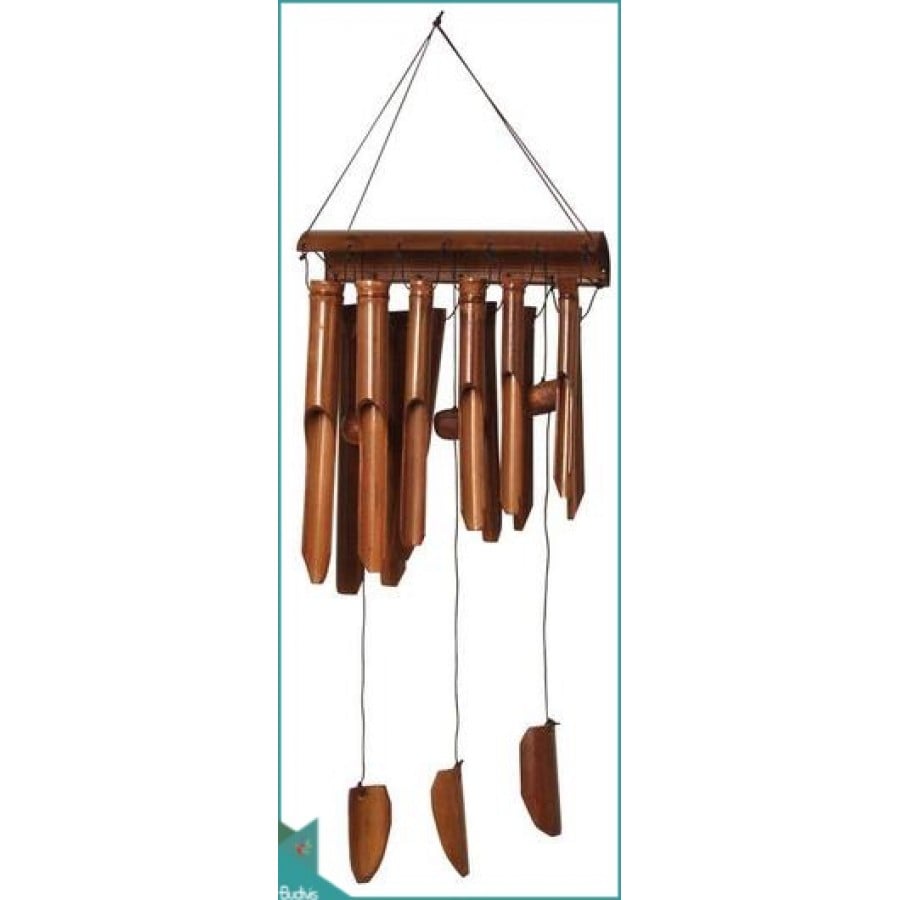This is a digitally created or hand-drawn image of a set of wind chimes against a white background. The wind chimes are arranged in a rectangle frame, with the tallest chime on the left and progressively shorter chimes towards the right, totaling six chimes. Each chime is suspended from a wooden fixture by strings that connect to a single hook at the top. Below the wooden fixture, three additional strings hang down, each with a small round wooden clapper designed to strike the chimes and make noise. The background is predominantly white with a pale aqua or teal rectangular border around the wind chimes. The wind chimes and their components appear to be either brass or wood, featuring colors like light brown, brown, teal, black, and white. There is a logo in the lower left corner of the image. The design suggests a balance with equal spacing around the elements, emphasizing the chimes as the focal point.